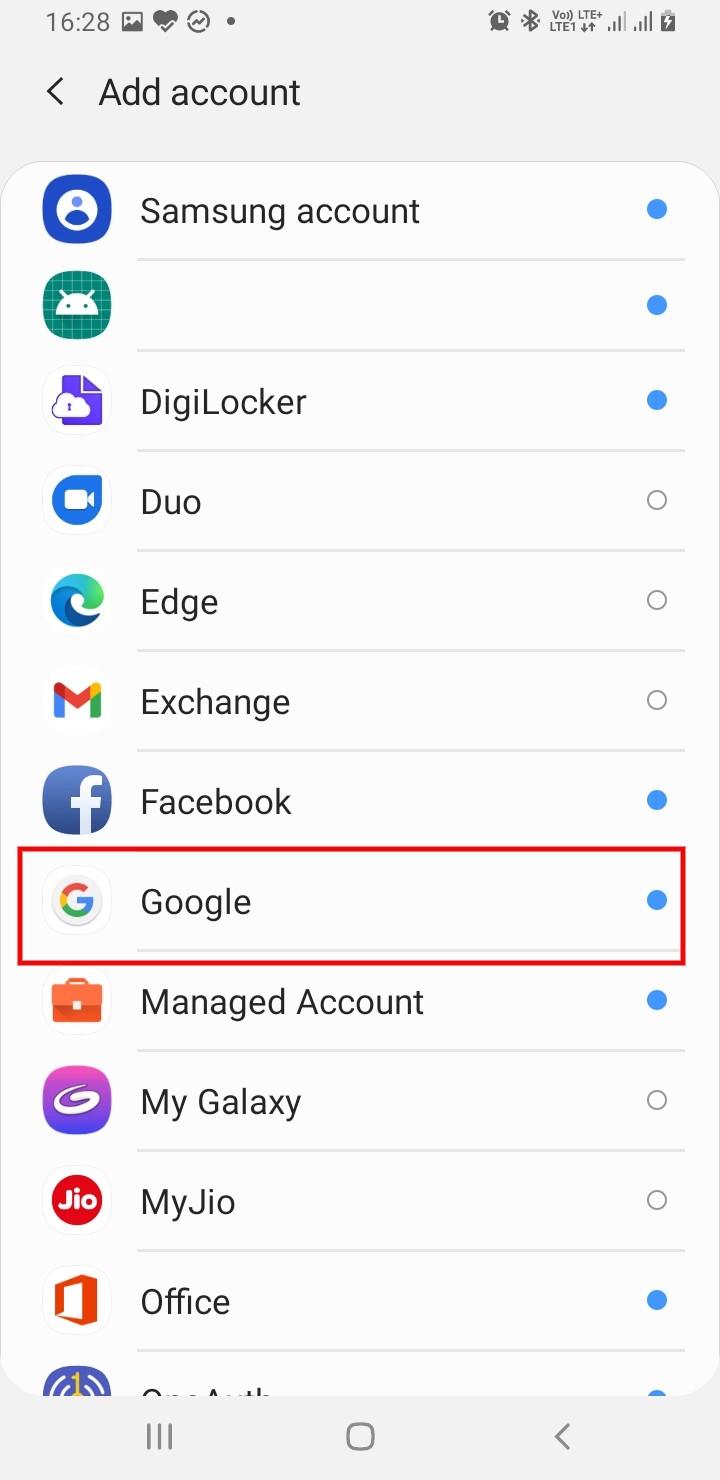In this image, we see a detailed screenshot of a mobile device interface. In the top-left corner, the time is displayed as 16:28, indicating it is 4:28 PM. Below the time, we observe various app icons such as the Health app, the Photos app, and others. Moving to the top-right corner, there are several status icons, including an active alarm icon, Bluetooth icon, VoLTE (Voice over LTE) icon, signal bars for two SIM cards, and a battery charging icon.

The main part of the screen showcases a variety of app icons and accounts. These include an ad account, Samsung account, DigiLocal, Duo, Edge, Exchange, Google Exchange or Gmail Exchange, Facebook, Google, a managed account, My Galaxy, My Geo, and Office. At the bottom of the screen, the navigation buttons are visible: the Recent Apps button, the Home button, and the Back button. This comprehensive setup provides a detailed view of the user's mobile interface and active applications.